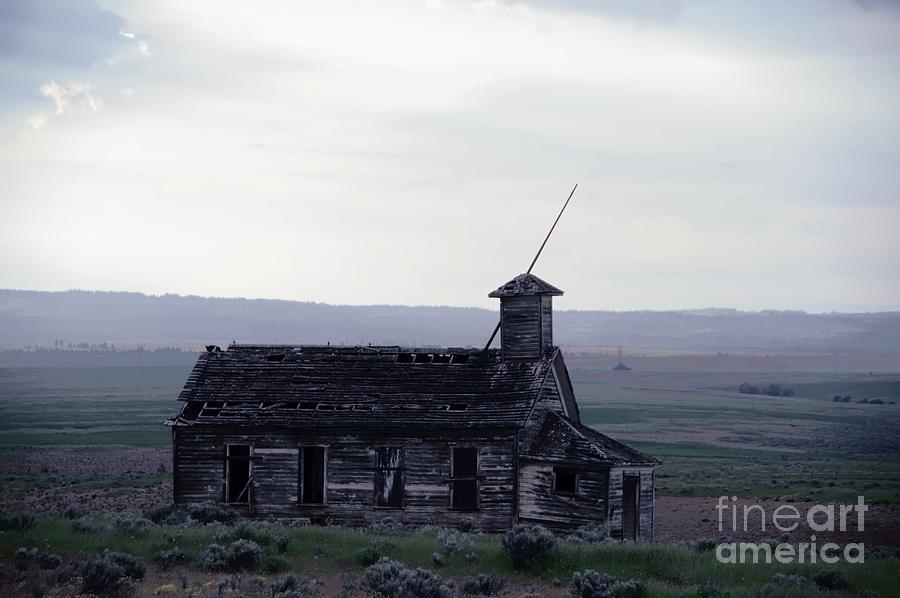This photograph captures an old, dilapidated wooden building, seemingly from the old western period, standing in isolation on a vast prairie. The structure is worn-down with holes in the roof and dark, mildew-streaked wood. The one-story building features four tall, rectangular windows along its side and an offset entryway with a smaller roof of its own and a single door. There is a curious addition on top that could be a steeple or a bell housing. The roof appears partially collapsed.

The prairie around the building is a mix of brown and green hues, dotted with wild weeds, bushes, and small trees. In the background, the flat land gives way to a ridge or a slight elevation change, though not quite mountainous. The sky above is mostly white with wispy clouds and hints of blue, indicating broad daylight. A watermark reading "fine art america" is visible in the lower right corner.

The scene is eerily serene, depicting an abandoned structure that might have once been a schoolhouse, church, or farmhouse, now left to the whims of time and nature. The setting hints at either spring or fall, adding to the nostalgic feel of this solitary relic on the prairie.